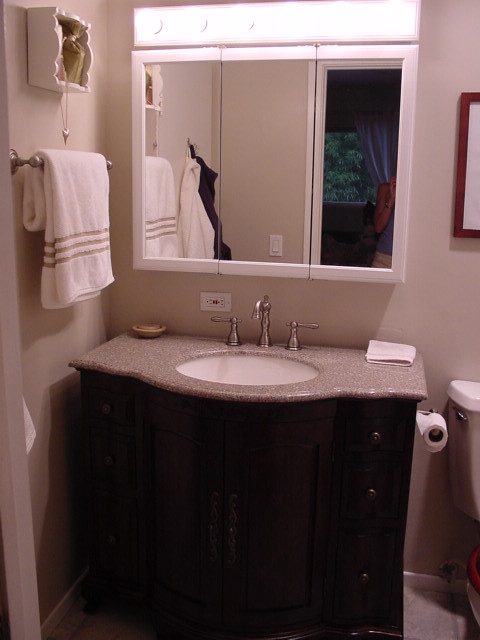A dimly lit bathroom-focused image, showcasing an elegant vanity area. The focal point is a three-piece, white-framed mirror mounted on the wall, illuminated by a rectangular strip of circular white light bulbs reminiscent of vintage dressing room fixtures. The sink area features a stone countertop with polished silver fixtures and a white basin, set in a dark brown wooden dresser-like stand adorned with metal handles. To the far right, the image subtly captures the edge of a white porcelain toilet. Adding to the decor, a white towel with gold striping hangs neatly on a brass-looking towel holder affixed to the wall. The soft lighting creates a serene atmosphere, casting gentle shadows that obscure some wall details.